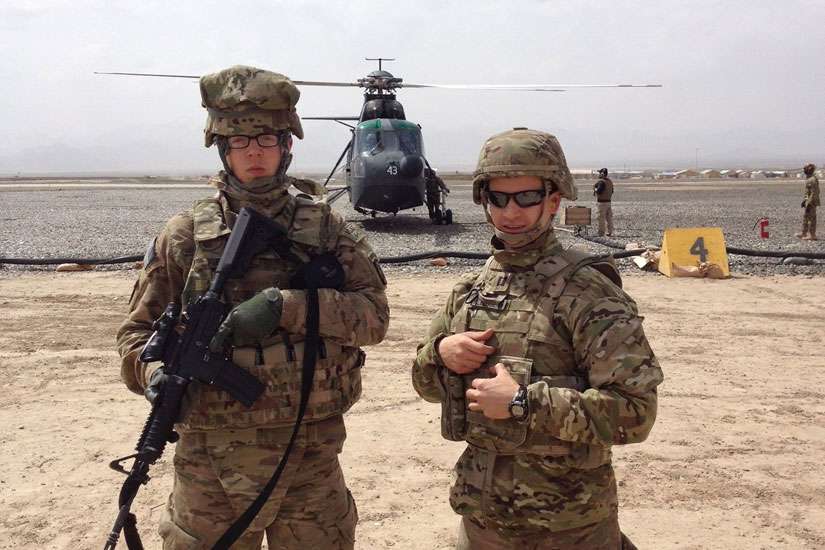This photograph captures two young, Caucasian male soldiers in a desert setting, with a Black Hawk helicopter poised in the background, ready for takeoff. The soldiers, possibly from the army or marines, are clad in full military fatigues, including helmets. The soldier on the left, who is holding a machine gun pointed downwards, wears prescription glasses and gloves. In contrast, the soldier on the right sports sunglasses and is unarmed, with his hands ungloved. Hovering over a ground that transitions from sandy dirt in the foreground to gravel in the background, the helicopter frames the scene under a gray sky. A yellow placard with the number '4' and the helicopter's nose marked with '43' adds a detailed touch, possibly indicating the landing area.